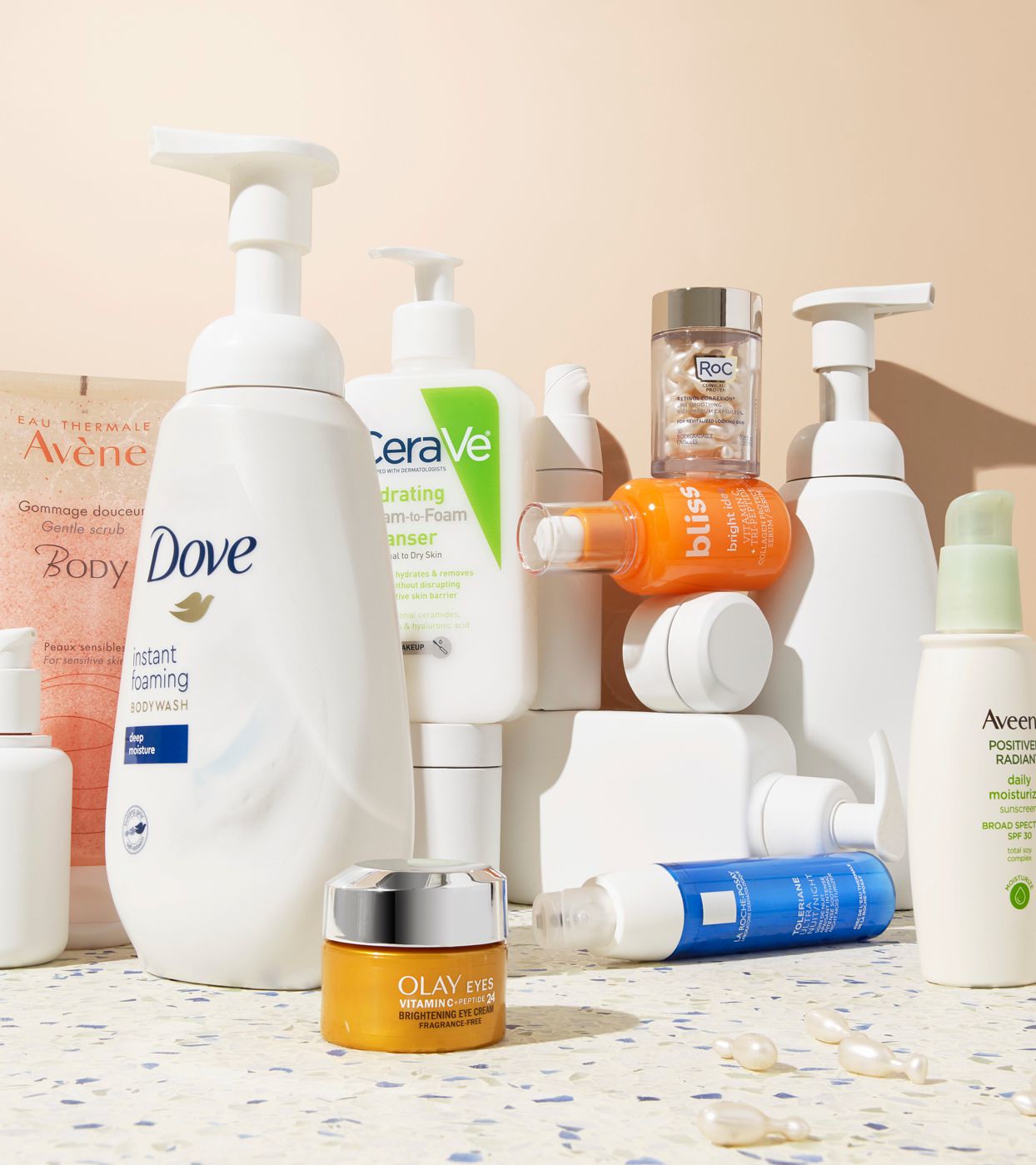This photograph captures an assortment of skincare and beauty products arranged on a ceramic-tiled countertop, set against a cream-colored wall. The subtle gradient on the wall transitions from lighter tones on the left to darker hues on the right. Positioned centrally but slightly towards the right, there is noticeable shadow play from one of the pump bottles.

Starting from the left side, the scene begins with a small, unlabeled container. Behind this is a pink tube standing upright, clearly labeled "Eau Thermale Avene Gommage Douceur Gentle Scrub Body." Adjacent to it is a substantial white pump bottle of "Dove Instant Foaming Body Wash."

In the foreground, there’s a small jar of Olay Eyes Vitamin C Peptide Brightening Eye Cream, notable for its mustard-colored jar and silver lid. Behind this, there's a partially visible white jar supporting a plastic pump bottle identified as "CeraVe Hydrating Foam to Foam Cleanser." This product is specifically noted for dry skin.

Moving right, there is a white bottle without a label, positioned atop another sideways white pump bottle, also unlabeled. In front of these, laying on its side, is a "La Roche-Posay Toleriane Ultra Nuit" night cream, recognizable by its clear white lid.

In the bottom right corner of the image, there appear to be peptide capsules, small in size and containing an oil inside, typically used daily. Above these, an orange bottle labeled "Bliss Bright" lies on its side, featuring a clear lid atop its pump area. 

Further right, a clear jar with a silver lid, likely storing the peptide capsules mentioned earlier, sits atop a container marked “ROC.”

On the far right side, another white pump bottle without a label stands, and beside it is the "Aveeno Positively Radiant Daily Moisturizer with Broad Spectrum SPF 30," easily identified by its green plastic pump dispenser.

Overall, the photograph meticulously showcases a variety of skincare essentials, each contributing to a visually interesting and coordinated display against a softly hued background.